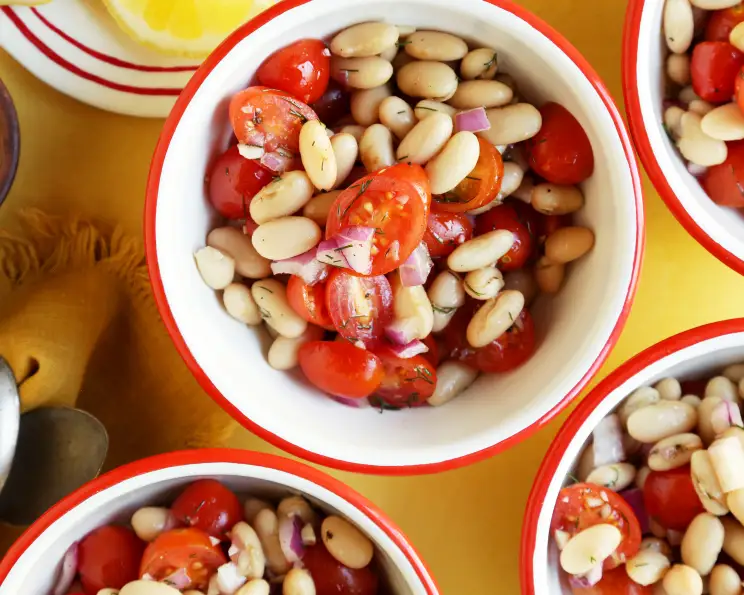This is an overhead, indoor color photograph showcasing a vibrant food arrangement. At the center lies a small, white ceramic bowl rimmed in red, filled with white beans, likely navy beans, mixed with chopped cherry tomatoes, red onions, and possibly pimentos. The colorful ingredients, with the glossy appearance of the pimentos and rich red of the tomatoes, are arranged in a visually appealing manner. Surrounding this centerpiece are partially visible identical bowls with the same contents. A hint of herbs can be spotted amongst the ingredients, adding to the fresh and appetizing look. All the bowls rest on a yellow tablecloth, adding a bright background to the scene. To the top left, a white plate with red stripes holds a slice of lemon, partially obscured from full view. The overall composition is colorful and delicious-looking, enhanced by the clear, focused photography.